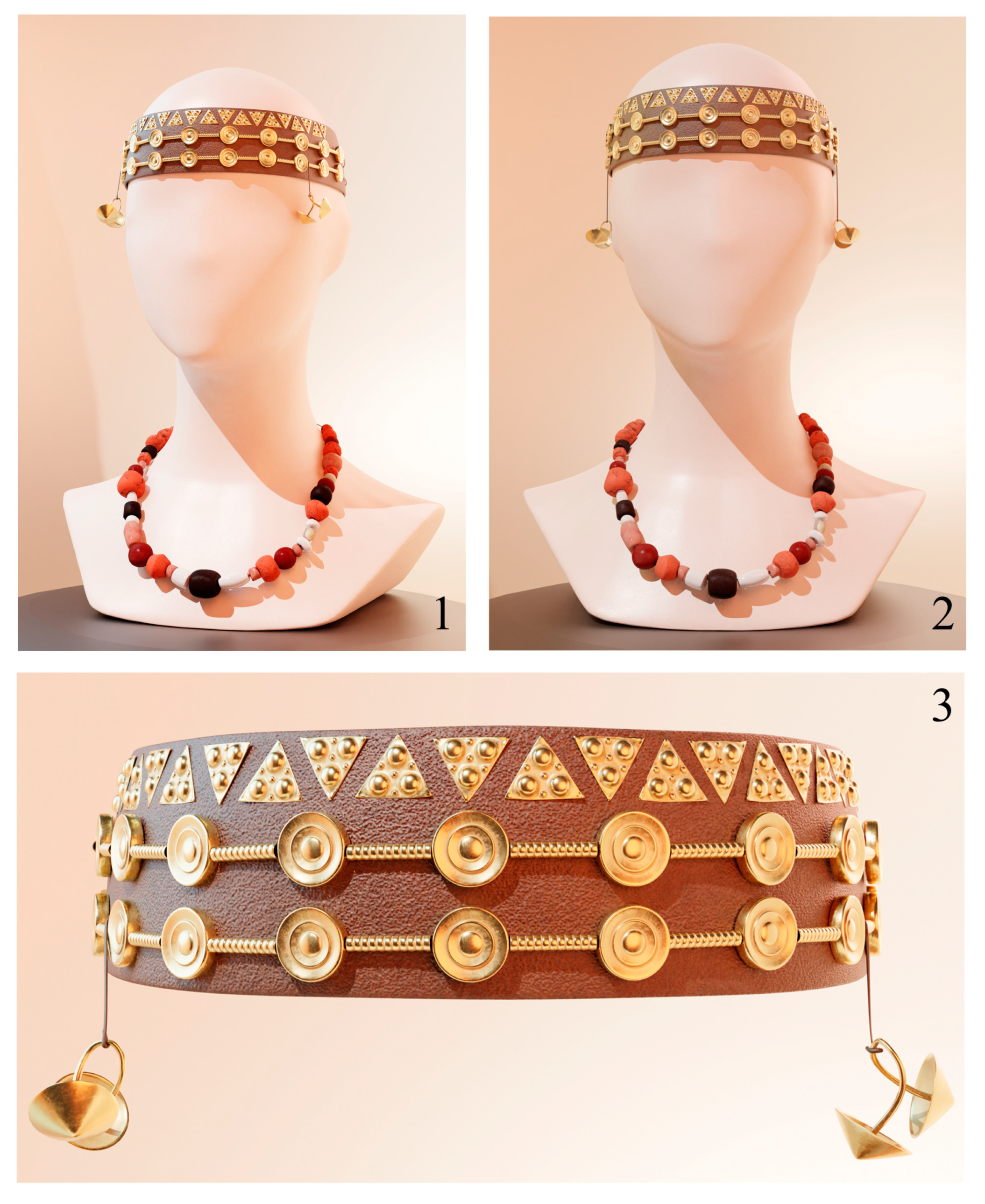This image is a triptych consisting of three frames, arranged with frames 1 and 2 side-by-side at the top, and frame 3 horizontally at the bottom. Each frame features the busts of mannequins adorned with a detailed headband and necklace, except the last frame, which focuses solely on the headband. 

**Frame 1:** Depicts a mannequin's head turned towards the left, showcasing a headband made of leather intricately beaded with gold embellishments. The headband features small dangling chains, detailed with gold beads. The mannequin wears a necklace with large clay beads in shades of pink, white, and black.

**Frame 2:** Displays a front-facing mannequin with similar adornments as in frame 1. The headband’s two dangling chains hang more towards the ears, complementing the flat-eared mannequin. The necklace remains prominently beaded.

**Frame 3:** Offers a close-up view of the headband. It reveals finer details: a leather band adorned with gold beads and chains, highlighting the careful craftsmanship. The absence of a mannequin draws attention entirely to the ornate headgear.

The major colors featured in the images are brown, gold, black, red, and various shades of white, complementing the intricate design and luxurious feel of the accessories. The wooden surface and the overall composition emphasize an elegant presentation without any textual distractions.